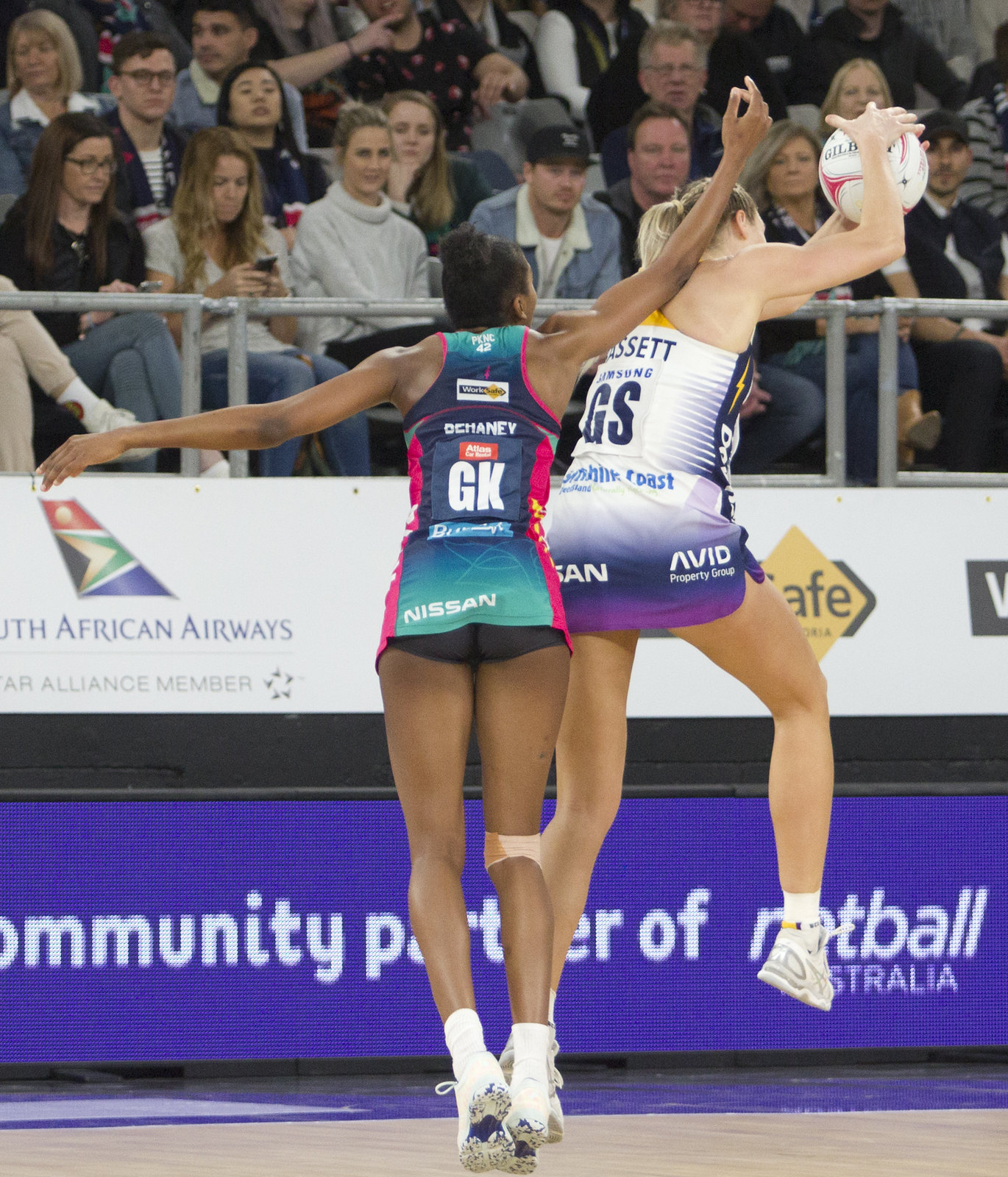In this vibrant and dynamic photograph, two women are captured in the midst of an intense volleyball match. Dominating the center of the image is a woman with brown skin and brown hair tied up in a bun. She is wearing white shoes and white socks, black shorts, and a colorful tank top with various logos including Nissan on the back, indicating she is likely the player named O'Chaney GK. She is depicted from behind, mid-jump, reaching with her right hand towards her opponent.

To her left and slightly ahead is her blonde opponent, sporting a tank top predominantly white and purple with logos such as Samsung and SSETT, and pink short shorts with "Avid" visible at the bottom. She is also mid-jump, holding the white and red volleyball with both hands. The blonde player’s energetic leap propels her toward the right side of the frame, highlighting the athleticism of the moment.

In the backdrop, an enthusiastic crowd is visible behind a metal railing, intently watching the unfolding action. Below the audience, advertisements including prominent names like South African Airways are displayed on a digital board, adding to the bustling atmosphere of the arena. The imagery and attention to detail vividly capture the spirit and excitement of the sporting event, complete with subtle nods to the community sponsors involved in the game.